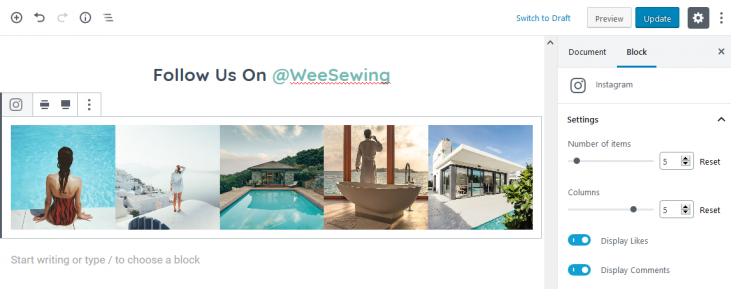This appears to be a screenshot of a user interface, likely from a content management or social media design tool, displayed on a screen with a white background.

At the top, there is a gray toolbar featuring several icons: a gray circle with a gray plus sign, an undo button, a redo button, an information icon, and three slightly staggered horizontal lines, all in gray. To the right of these icons, there is blue text reading "Switch to draft." Next to this, there are multiple buttons: a light gray button with darker gray text that says "Preview," a blue button with white text that says "Update," a dark gray button with a white gear icon likely representing settings, and three vertical gray dots which probably open a menu.

The main window of the display is showing an image being edited, with a header that reads "Follow us on @we_sewing." Below this header, there is a gray box containing five images of various vacation locations. Above this gray box, there is a camera icon and another icon which might be a print option or alignment tools. The bottom of the main window features gray text prompting the user to "Start writing or type / to choose a block," which indicates this area is for content creation.

In the sidebar on the right, under the header "Document," there is a tab named "Block," which is selected and indicated by a bold label with a blue underline. Adjacent to this is a close button. Below these tabs, there is a camera icon labeled "Instagram," followed by a light gray line separating this from additional settings. These settings include "Number of items" with a slider bar and a box set to five, which includes up and down arrows beside it and a "Reset" button. There is another setting for "Columns" with similar controls. Further down the sidebar, there are two blue toggles: one labeled "Display likes" and the other "Display comments," both of which are selected (ON).